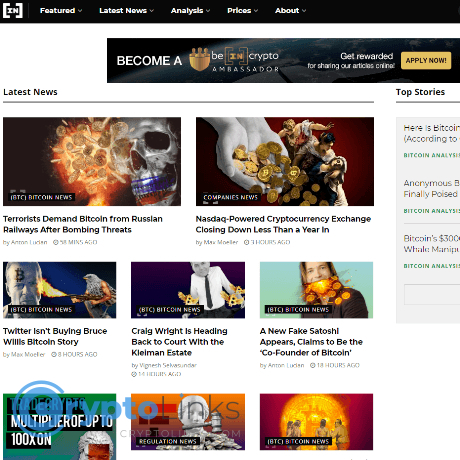The image depicts a cryptocurrency news website with a sleek, user-friendly design. 

At the top, there is a black navigation bar featuring the white letters 'XN'. This navbar includes drop-down menus for 'Features', 'Latest News', 'Analysis', 'Prices', and 'About'. Directly below this navigation bar, a prominent black banner displays a call to action: "Become a Crypto Ambassador" with an "Apply Now" button.

Below the banner, the website is divided into two main sections. On the left, occupying approximately 80% of the space, is the 'Latest News' section. This section showcases three rows of news posts. The top row features two large images with headlines: "Terrorists Demand Bitcoins from Russia Railways after Bombing Threats" and "Nandex-Powered Cryptocurrency Exchange Closing Down Less than a Year In." The bottom two rows each contain three smaller images with news headlines.

To the right of this 'Latest News' section and below the banner, there is a 'Top Stories' segment, which lists three stories, though the majority of this information is cut off in the image. The website's overall layout focuses heavily on presenting recent and critical news in the cryptocurrency sphere.